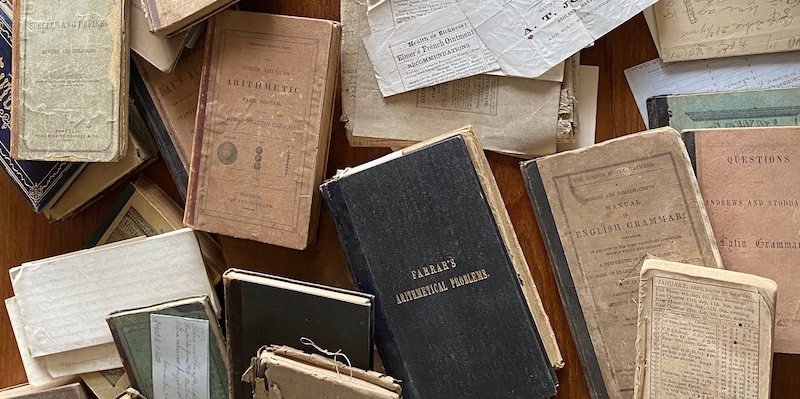This image depicts an assortment of very old books and loose papers scattered haphazardly across a warm, dark wooden table. The surface of the table is barely visible beneath the chaotic array of items. The collection includes a variety of both paperback pamphlets and hardcovers, with the latter predominantly in black.

One of the most prominent books occupies the bottom middle section of the image, slightly askew, and bears the title "Faraz's Arithmetical Problems" in faded gold lettering on a black cover with a hint of the spine showing tattered pages. Other notable titles include "A Manual of English Grammar," another book on arithmetic, and a book titled "Questions" with the subtitle "Latin Grammar."

Amid the books, there are scattered loose pages, some folded, with handwritten notes. At the top middle section, loose papers appear to have fallen from a book. One of the pages features the term "health" and highlights "Elmer's French Ointments." Another page seems to be a monthly planner with "January" and a list of dates and numbers. The overall arrangement of the items suggests a sense of age and well-worn use, with pages sticking out at odd angles and some covers missing entirely.